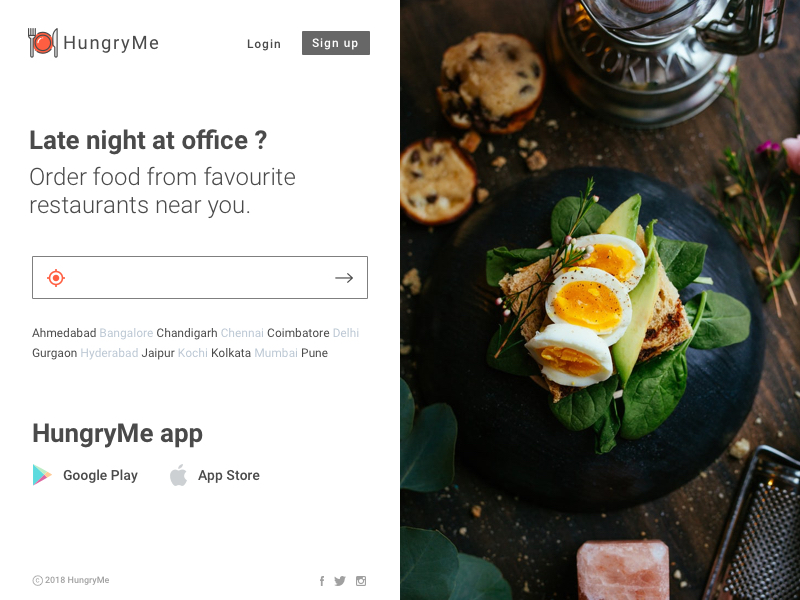This is a detailed caption for the given screenshot of the website "Hungry Me":

The screenshot captures the homepage of the website "Hungry Me." At the top, two prominent options are displayed: "Log In" and "Sign Up." Beneath these options, a headline reads, "Late night at the office? Order food from your favorite restaurants near you." Just below this text, a location input box is prominently featured, allowing users to search for nearby restaurants. Underneath the search box, a series of popular restaurant choices is shown, likely representing frequently selected options by users.

On the right side of the screen, there is a visual enticing users to explore the Hungry Me app, available on both Google Play and the App Store. Additionally, icons for social media platforms Facebook, Twitter, and Instagram indicate the website's presence on these networks.

A delectable image accompanies the webpage layout to the right. The image features two muffins stacked atop each other, surrounded by crumbs, alongside a third muffin. Next to the muffins is a plate showcasing a variety of green leafy vegetables, likely spinach, with an avocado-topped bread or sandwich. The plate also includes three egg halves: two halves from one boiled egg and another single half egg nestled amongst the greens. The table settings include what appears to be a metal kettle in the top corner and various flower stems, enhancing the visual appeal of the scene.